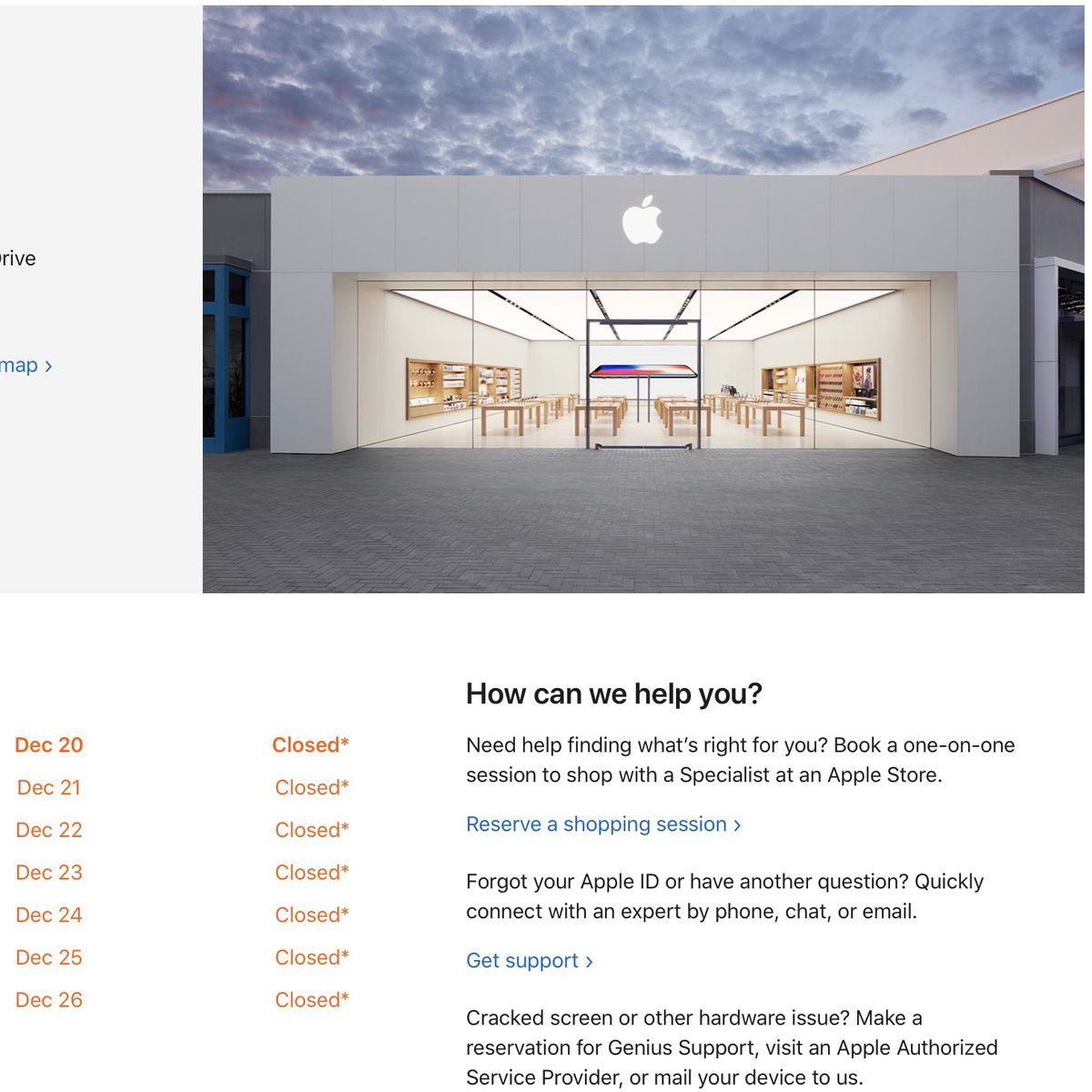The image depicts a closed Apple Store at dusk, under a cloudy sky. The storefront is distinctly white, with the glowing Apple logo prominently centered. The building's entrance is entirely glass, offering a clear view of the interior. Inside, several wooden tables are neatly arranged, flanked by built-in displays and shelves made of the same light-colored wood.

To the side of the image, there's a partially visible gray informational box. It lists dates between December 20th and 26th, all marked as "closed," with the 20th highlighted in bold and accompanied by asterisks for each "closed" entry.

On the left side of the screen, a bold black heading reads "How can we help you?" Below this, text invites customers to book a one-on-one session with a specialist at an Apple Store via a blue hyperlink saying "reserve a shopping session." Further down, the text in black asks if you have forgotten your Apple ID or have other questions, directing you to connect with an expert by phone, chat, or email through another blue hyperlink labeled "get support." Additional information in black advises on how to address cracked screens or other hardware issues by making a reservation for Genius Support, visiting an Apple authorized service provider, or mailing your device for service.